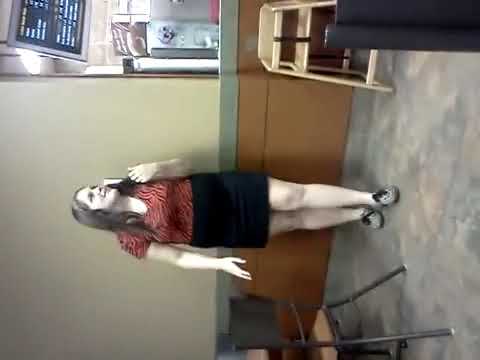The image features a woman standing in what appears to be a cafe or a corner of a restaurant, with the photograph rotated 90 degrees to the left. She is standing on a blue-brown floor against an olive green wall with brown paneling below. Her outfit includes a black skirt that goes above her knees and an orange and black striped short-sleeved top. She has medium brown hair that falls past her shoulders, and she is seen touching or playing with it with her left hand while placing her right hand on her waist. The woman, who has white skin, is gazing towards her left, which would be upwards in the rotated photo. On her feet, she wears gray shoes with black shoelaces, though another description mentions black and white sneakers. To her left is a chair, and to her right is a wooden high chair, suggesting the setting could be a restaurant or coffee shop. The background contains what might be a mural or menu board depicting a barista or a coffee machine. Above this, there appears to be a monitor with some text, indicating it could also be part of a cafeteria or a similar setting.